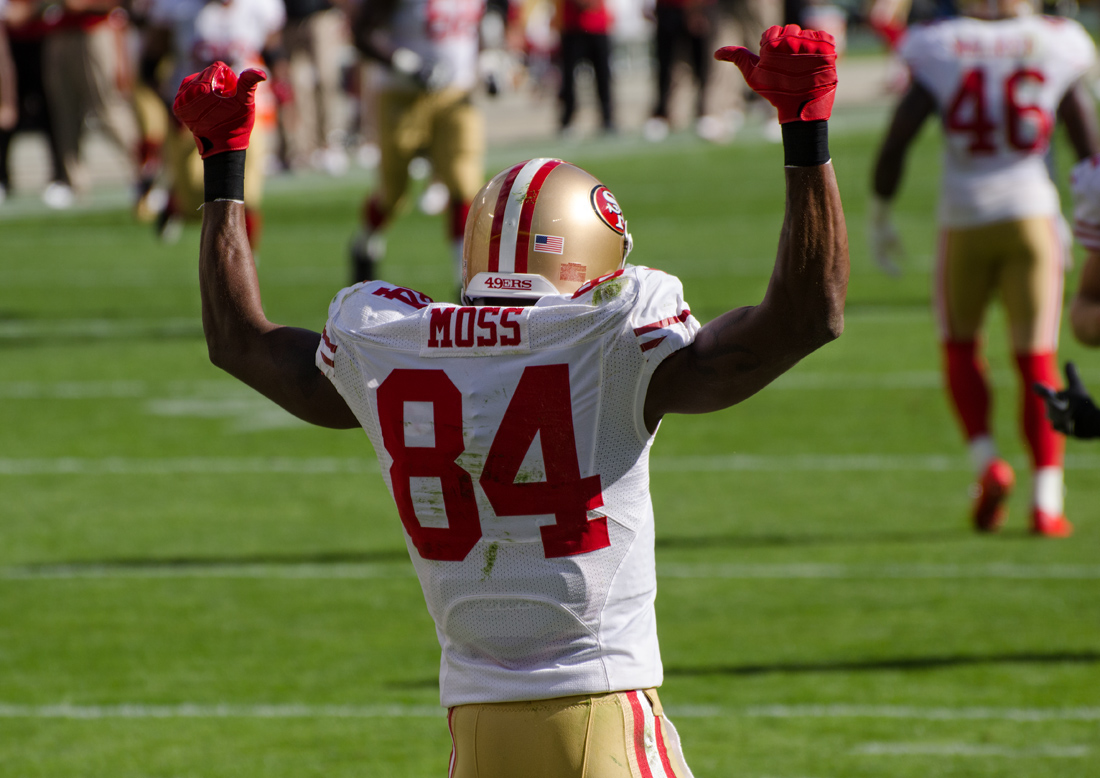The image captures a vibrant, daytime scene of a San Francisco 49ers football game. At the forefront is a black male football player, visible from the waist up, facing away from the camera with his arms raised. He is wearing a distinctive white jersey with red and gold accents, prominently featuring the name "Moss" and the number "84" in bold red letters on the back. His uniform includes gold pants with white and red stripes along the sides, and red gloves on his raised hands. A gold helmet adorned with a white and red stripe and the SF logo sits atop his head. The action takes place on a green football field marked with white lines and numbers, with other 49ers players and individuals on the sidelines visible in the blurred background, suggesting a bustling, lively game setting captured in clear, natural daylight.